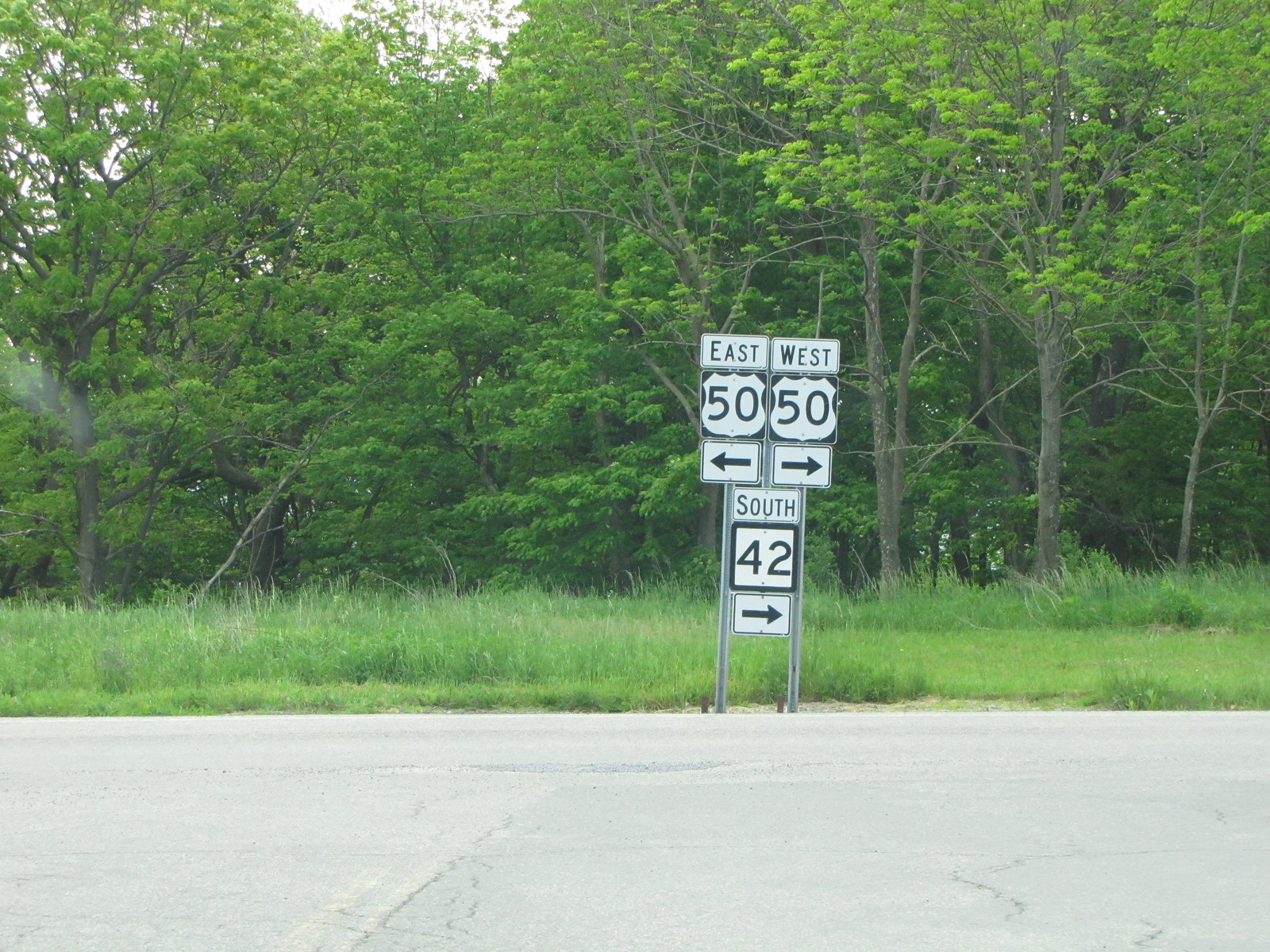The image showcases a directional sign situated at the end of a slightly cracked and weathered road, captured straight-on from a distance. The faded central line of the road is nearly indistinguishable, appearing more as a subtle indentation than a defined marker. To the side of the asphalt, a stark contrast in grass height is visible; on one side, the grass is noticeably tall and unkempt, while on the other, it is trimmed low. This grassy area transitions into a dense backdrop of green, leafy trees, reflecting a vibrant spring or summer season.

The sign itself is mounted on a metal pole and contains clear directional arrows: one designates "East-West Route 51," while another indicates "Route 50" in the opposite direction. Additionally, an arrow points southward, marking "Route 42." The scene overall evokes a sense of rustic, countrified tranquility amidst overgrown nature and well-trodden paths.